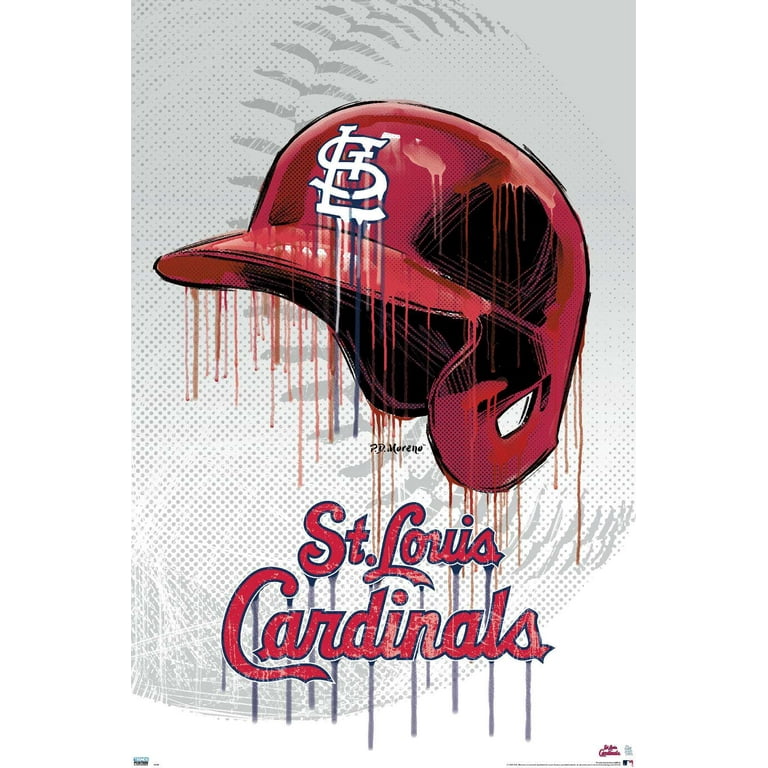This painting presents a stylized depiction of a St. Louis Cardinals batting helmet, vividly red and distinct with the iconic "STL" logo in white on the front. The helmet appears as if fresh paint is dripping off it, creating a melting effect with streams of red running down the sides and bill. Behind it, a soft gray background features a speckled design resembling a baseball, with visible gray stitching at the top left and bottom right corners of the image. Below the helmet, scripted lettering with a red fill and black outline reads "St. Louis Cardinals," also exhibiting a melting or dripping effect that ties together with the helmet's artistic representation. The overall composition emphasizes a visual merging of elements, giving the impression of motion and fluidity in the traditionally static symbols of baseball.